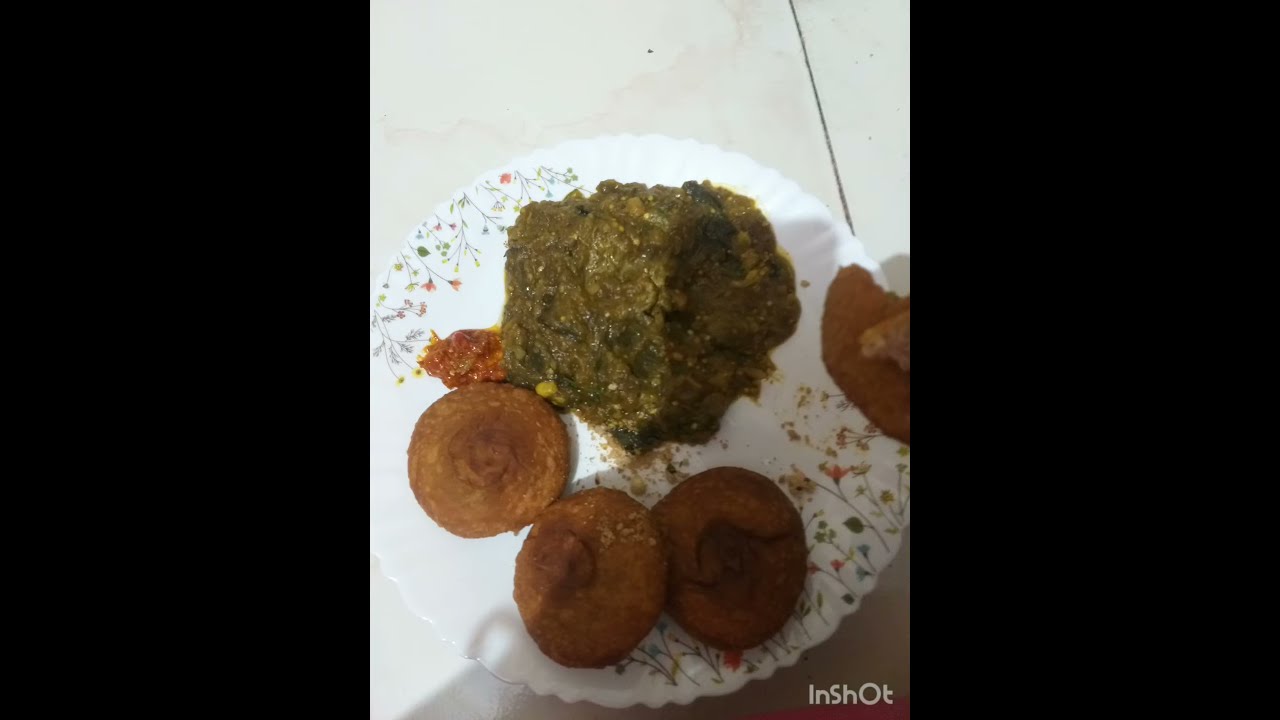The image features a top-down view of a white, scallop-edged plate adorned with a delicate flower design, incorporating small, stemmy flowers in red, pink, blue, yellow, and green. This plate, on what seems to be a white surface with a distinctive black stripe suggesting a wooden table with visible slats, showcases a variety of Indian cuisine. Prominently, there is a portion of saag, a traditional spinach dish. Accompanying this are three brown, disc-shaped items, likely fried plantains or potatoes. Additionally, a small serving of red sauce is present near these discs. The overall composition of the tableware and food elements is well-defined against the white background, with shadowy areas towards the bottom of the image.